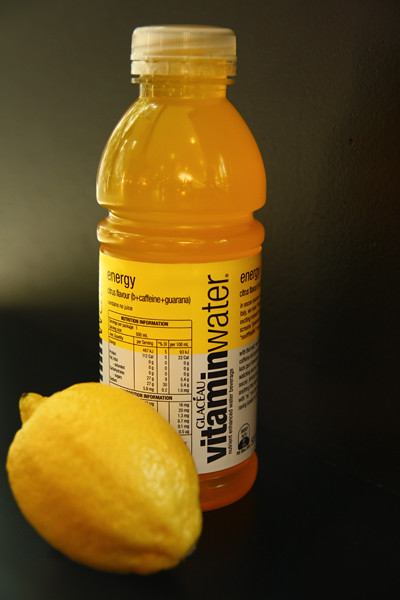This high-quality photograph showcases an unopened bottle of yellowish-orange Vitamin Water, approximately 16 ounces, in its original plastic packaging with a white wrapper and the word "energy" visible on it. The bottle is positioned to display the nutritional information and ingredients. In front of the bottle is a whole, uncut lemon, suggesting a possible lemon flavor for the drink. The background is predominantly a dark, slate gray, with some light hitting parts of it, particularly in the upper half of the image, while the bottom half remains darker. Additionally, there seems to be some text or markings along the left edge of the photo. This scene evokes a sense of care, akin to leaving a Vitamin Water and lemon for someone feeling under the weather.